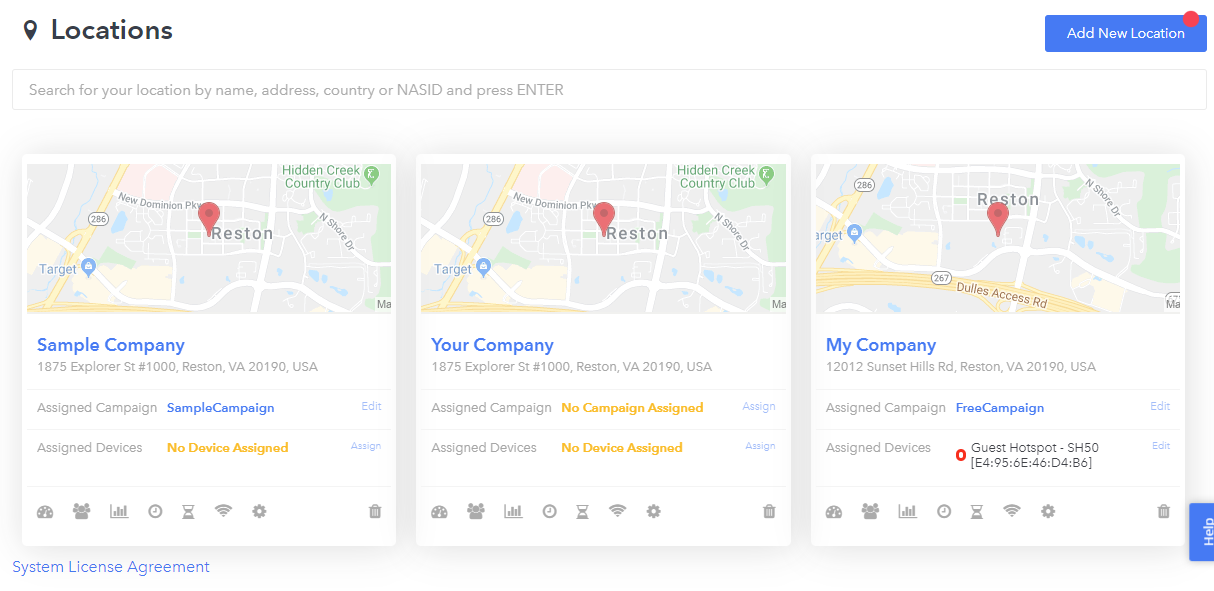This screenshot displays an interface for managing different locations within a campaign management system. At the top left of the screenshot, the section is labeled "Locations" and features a search bar below it, intended for users to search for a location by name, address, country, or "nest seed," with an instruction to "press enter" after inputting the query.

On the top right of the screenshot, there is a prominent blue button labeled "Add New Location" in white text. Additionally, a red notification dot is visible at the top right corner, presumably indicating new or pending actions.

Below this header area, three location entries are displayed side-by-side:

1. **Sample Company (left section)**:
   - **Address**: 1875 Explorer Street
   - **Assigned Campaign**: Sample Campaign
   - **Assigned Devices**: No assigned devices

2. **Your Company (middle section)**:
   - **Address**: 1875 Explorer Street
   - **Assigned Campaign**: None
   - **Assigned Devices**: No assigned devices

3. **My Company (right section)**:
   - **Address**: 1875 Explorer Street
   - **Assigned Campaign**: Free Campaign
   - **Assigned Devices**: Guest Hotspot